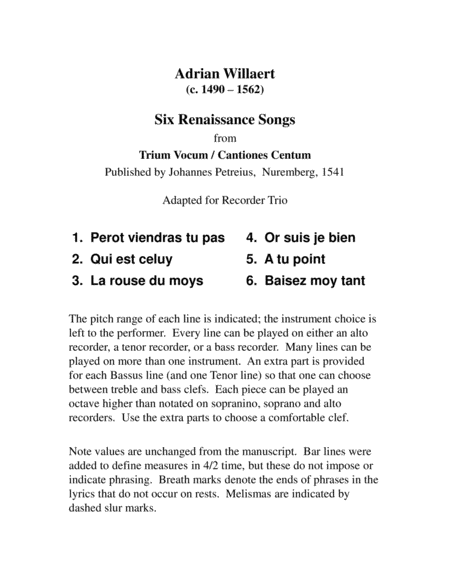This vertical image, which lacks an outside border, features black text on a white background and appears to list songs by Adrian Willard. The header reads "Adrian Willard, circa 1960 to 1962" followed by the title "Six Renaissance Songs" in darker print. Below this, smaller print details that the songs are adapted for a Recorder Trio. The six song titles listed are not in English. The text also states that the music is adapted from "Triumvokum/Cantione Centum" published by Johannes Petrius in Nuremberg, 1541. It outlines that the pitch range of each line is indicated, and that the instrument's choice—alto recorder, tenor recorder, or bass recorder—is left to the performer. Additionally, many lines can be played on more than one instrument. Extra parts are provided for each bass and one tenor line to allow a choice between treble and bass clefs. Each piece can be played an octave higher on sopranino, soprano, or alto recorders using the extra parts for a comfortable clef. Note values remain unchanged from the manuscript, but bar lines were added to define measures in 4/2 time. These do not dictate phrasing, which is instead indicated by breath marks at the ends of phrases, and melismas are marked by dashed slur marks.